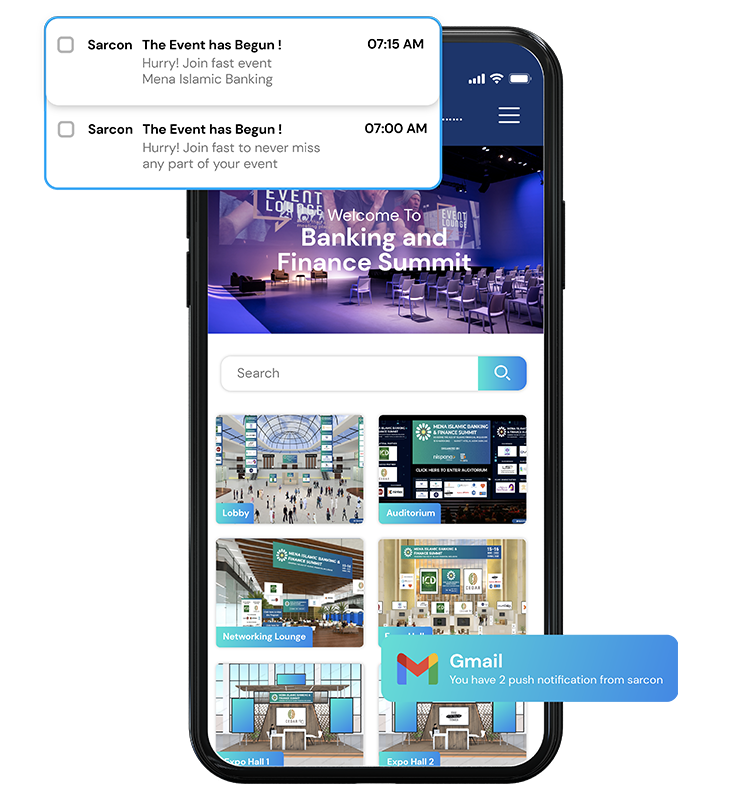The image depicts an Apple mobile phone displaying the interface for the Banking and Finance Summit. The phone screen showcases an image promoting the summit, followed by a search bar for easy navigation. Below the search bar, there are three rows of two images each, featuring various sections of the event, including the Lobby, Auditorium, Networking Lounge, Expo Hall 1, and Expo Hall 2. Overlaid at the top of the screen are push notifications simulating messages attendees would receive during the event. One notification reads, "The event has begun, hurry join fast - event: Mina Islamic Banking at 7:15 AM," while another, time-stamped at 7:00 AM, states, "The event has begun, hurry join fast to never miss any part of your event." Additionally, there are two push notifications from SACON, indicating incoming emails. This image effectively illustrates the interactive and informational features provided to participants of the Banking and Finance Summit.